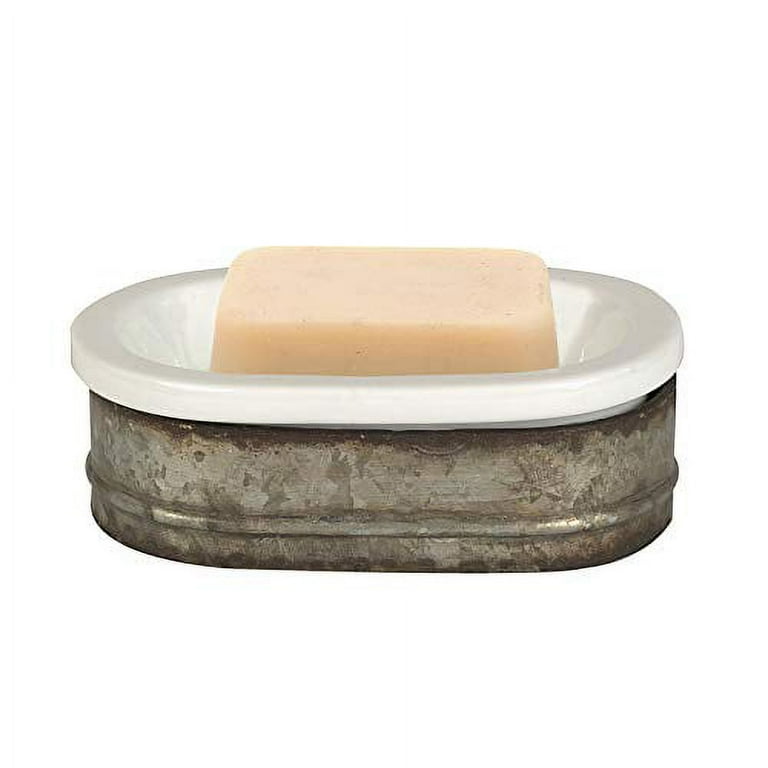The image showcases an old soap dish composed of a metal base and a white porcelain top. The metal base is round and has a rustic appearance with noticeable tarnish and splotches, including darker, rustier spots toward both the bottom and top edges. Nestled within this metal base, the white porcelain dish is smooth and oval, devoid of imperfections. Positioned in the center of the porcelain dish is a pristine, rectangular bar of soap with rounded edges. The soap is slightly peach in color, unblemished, and appears unused. The image is taken from the side, providing a clear long view of the entire soap holder structure in a pristine white background.